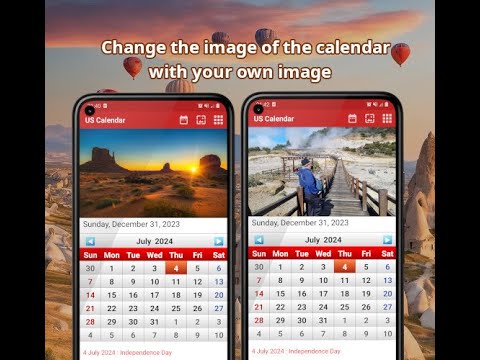This digital image illustrates how dynamic calendar customization works on mobile devices. It features two smartphones side by side, both displaying calendar apps for July 2024. The phone on the left highlights an "US Calendar" with a vivid desert scene under a shining sun, indicating a solitary, serene location. The screen shows detailed information such as the current date and time: Sunday, December 31, 2023. The calendar view is set to July 2024, with Thursday, July 4th, marked in red and labeled as "Independence Day." In contrast, the phone on the right exhibits a personalized calendar, featuring the image of a man standing on a wooden bridge surrounded by sandy terrain and lush green trees. This calendar also shows July 2024, with the same emphasis on July 4th as Independence Day. The overall message conveyed is the ability to modify calendar images to suit personal preferences, enhancing usability and personalization.